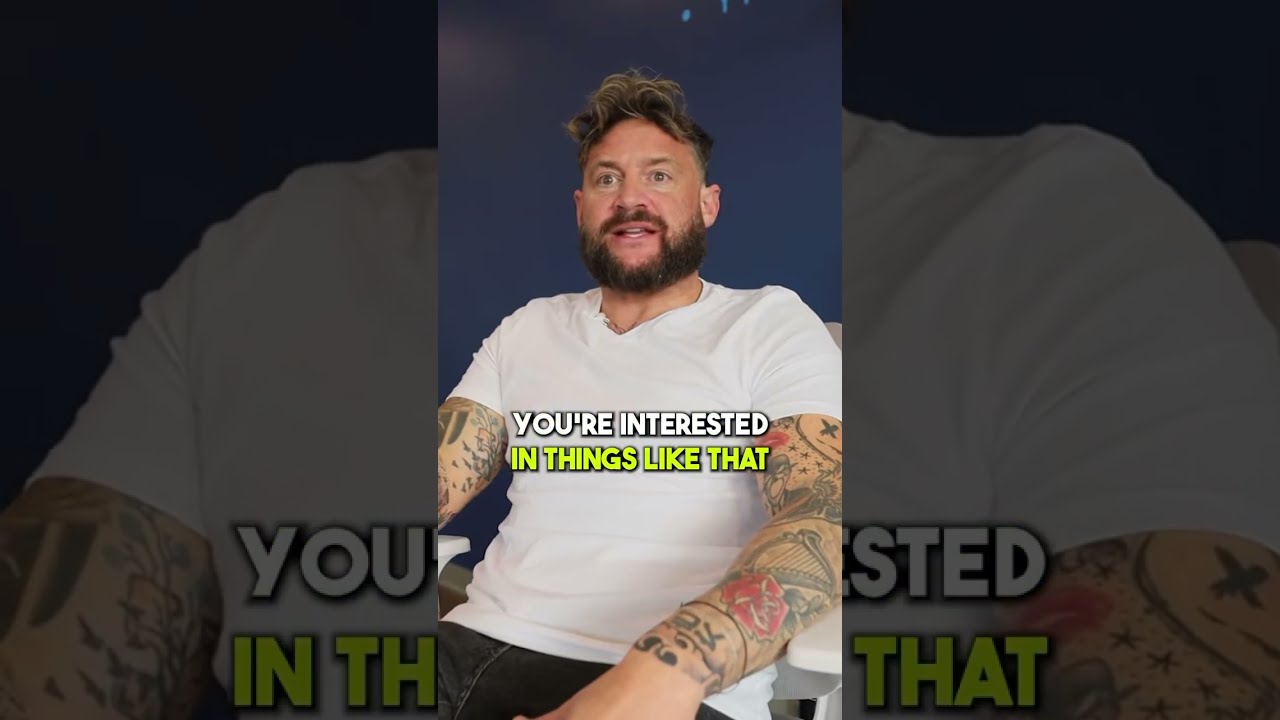A man is seated in a chair against a blue backdrop, seemingly in a video still that captures him in a mid-length portrait. He has a slightly agape mouth, giving him a look of surprise or contemplation. His hair is predominantly brown with some blonde streaks and appears somewhat wavy and disheveled. He sports a full brown beard. The man is wearing a plain white t-shirt, revealing his extensive tattoos that cover both arms in patterns of red, gray, and black. Though parts of his left arm are cut off from the image, the tattoos are still visible. He also has a wristband on his left hand. The image is bordered by a darker frame that shows more of his torso, including the top of his black jeans. Superimposed over his shirt is the bold, uppercase text that reads "YOU'RE INTERESTED" in white, and "IN THINGS LIKE THAT" in green, both framed by a border. The man appears to be of Caucasian descent and may have some visible tattoos or a necklace around his neck. His posture and the setup suggest he might be participating in an interview.